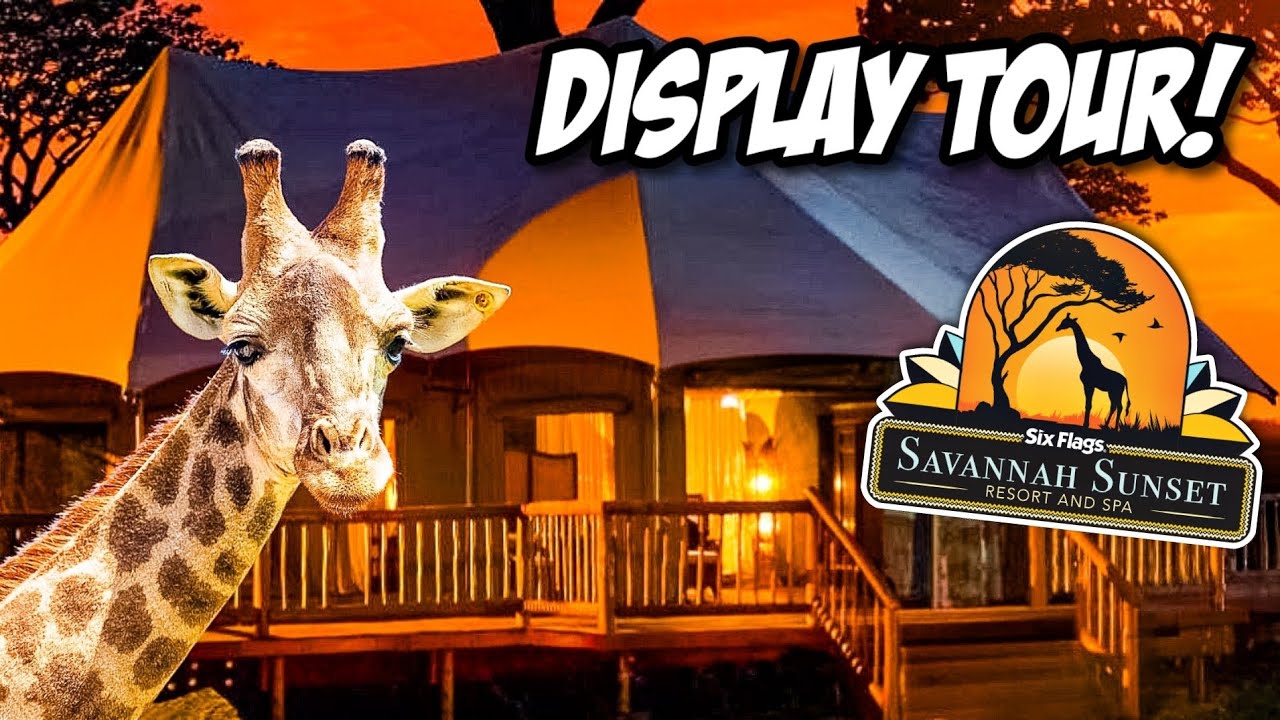The image is a vibrant advertisement poster, featuring a striking design that prominently showcases a giraffe peeking from the left side, appearing almost like a cutout. The background features a wooden structure with visible windows, a stairwell, and a canopy tent at the top, set against a mesmerizing orange sunset sky. The overlay text at the top in bold, white capital letters reads "DISPLAY TOUR!" Below this text is a logo depicting a safari scene with a large sun setting behind a tall tree, giraffe, and birds flying off to the right, in silhouette. The logo and accompanying text promote "Six Flags Savannah Sunset Resort & Spa," hinting at an adventurous, wildlife-themed getaway.